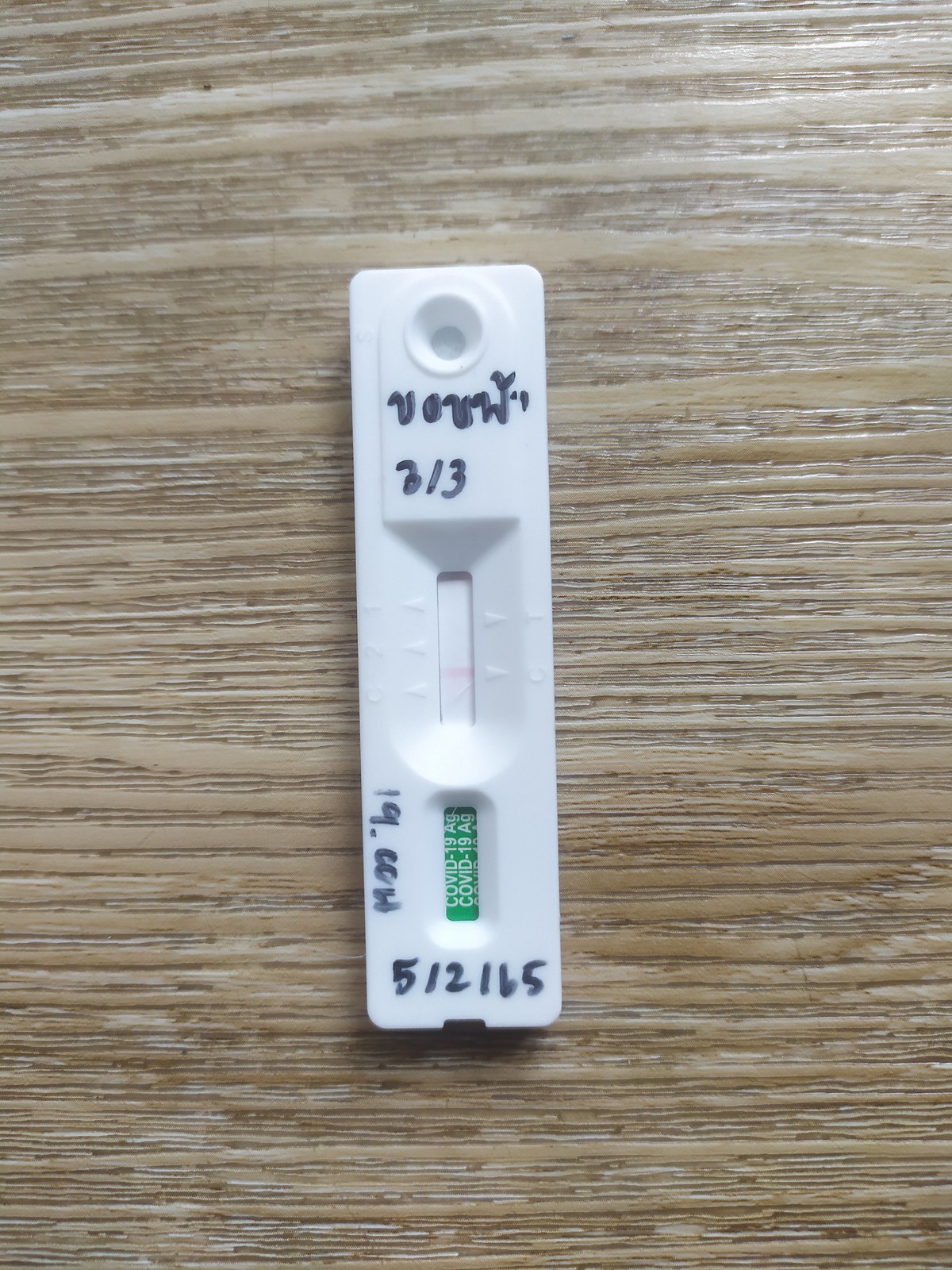The image showcases a close-up view of a desktop surface, which appears to be made from a brown, grainy wood, possibly walnut or oak. Resting on the surface is a white plastic COVID-19 test. The test device features a dropper depression at its top and a central litmus paper strip displaying a single pink stripe, indicating a negative result. Imprinted within an indentation on the test are the words "COVID-19 AG." A black Sharpie marker has marked a sequence that appears to read either "5-2-65" or "15." Additionally, along the left side of the test, there is an inscription reading "19 point something," though it is not entirely clear. Near the top of the test, there is a scribbled word, possibly in a different language, along with the numerals "3-3," which might denote March 3rd.